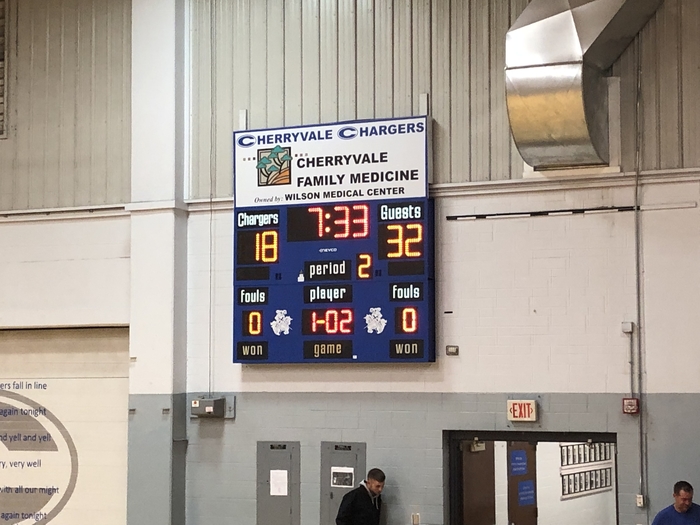This photograph, taken indoors, captures the interior of a gymnasium with its high, gray brick walls transitioning into white and then tan at the upper levels. The focal point of the image is an electronic scoreboard centered prominently against the backdrop. At the top of the scoreboard, "Cherryvale Chargers" is displayed in blue, and below that, it reads "Cherryvale Family Medicine," indicating sponsorship by Wilson Medical Center. 

The scoreboard details that the current time is 7:33 left in the second period, with the home team, Chargers, trailing at 18 points against the guests' 32 points. The fouls for both teams are displayed as 0 with additional information showing periods with 1 and 1 below. 

Two men, only partially visible from the chest up, stand adjacent to an open exit doorway at the bottom portion of the image. One man, wearing a black shirt, is on the left while the other, in a blue shirt, is on the right. Both men have brown hair. The photo encapsulates the atmosphere of a typical school gymnasium during a sporting event.